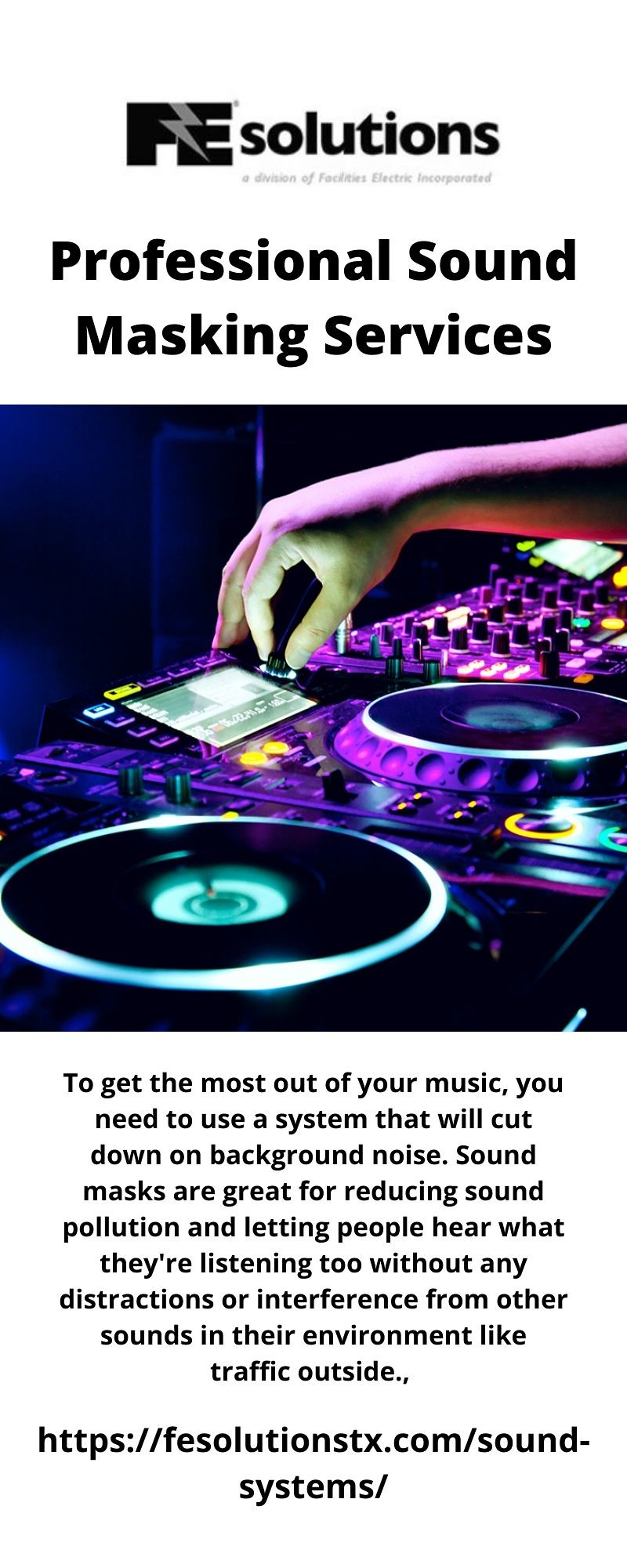This image appears to be a screenshot of an advertisement for FE Solutions, a company specializing in Professional Sound Masking Services. At the top, the company name "FE Solutions" is prominently displayed, with a lightning bolt that separates the "F" and "E." Beneath this, the tagline reads "Professional Sound Masking Services." The focal point of the image is a DJ's hand positioned over a turntable, reflecting neon colors from a lit-up soundboard that features a variety of dials, buttons, and digital screens. The vibrant scene includes accents of neon purple, green, and yellow, casting colorful reflections on the DJ's hand as they manipulate the controls. Below this visual, a synopsis explains that utilizing sound masking systems helps reduce background noise, allowing users to enjoy their music without interference from environmental sounds like traffic. The advertisement concludes with a URL for further information: https://fesolutionsstx.com/sound-systems/. All the text is presented in black.